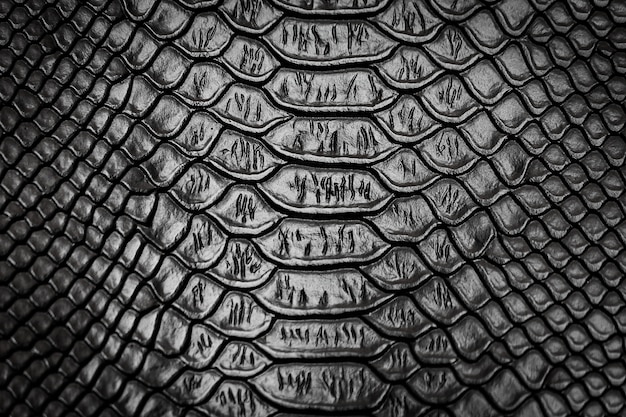The image is a highly detailed, close-up photo of dark, black snakeskin with a varied texture. The surface is covered with ridges and scales of different sizes, creating geometric patterns that stand out against the backdrop. The scales in the center of the image are the largest, gradually decreasing in size as they move towards the edges. These central scales have a smooth exterior but show visible markings or scratches, while the smaller scales on the sides are sleek and wrinkle-free, resembling lemon shapes. The lighting in the image is strategically placed, highlighting different shades of black and creating a reflective, almost silver appearance on some parts of the scales. The overall effect is a striking, textured pattern that captures the eye with its intricate details and subtle variations in light and shade.